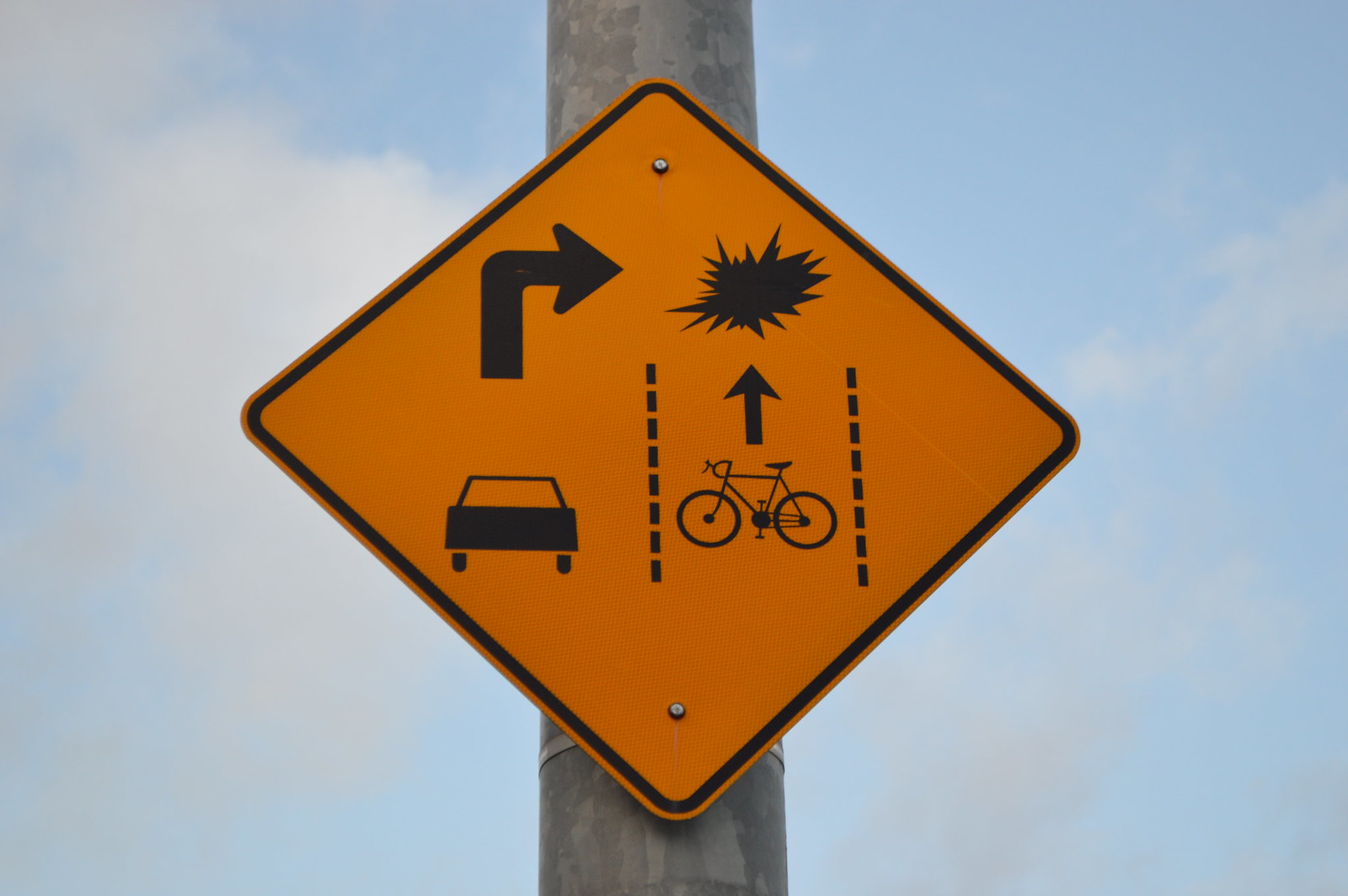This is a detailed photograph of a cautionary street sign affixed to a tall, weathered wooden pole, which shows various tans, beiges, and gray patches revealing its aged texture. The sign, a bright yellow-orange diamond with a black border, has silver rivets and gray straps securing it in place. It features a graphic depicting a car with a right-pointing arrow on the left, accompanied by dashed lines surrounding a bicycle with an upwards-pointing arrow and a symbolic crash or explosion image, indicating a potential collision. The scene is set against a backdrop of a mostly clear blue sky, accented by a few wispy white and gray clouds, giving a serene feel to the cautionary message. The sign serves to warn drivers making right turns to be mindful of cyclists continuing straight in the bike lane to prevent accidents.